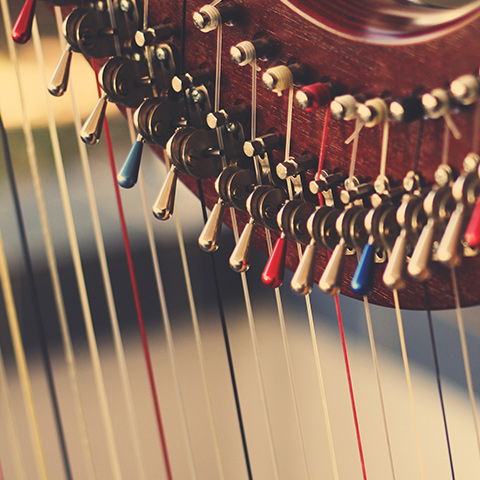The image is a high-quality, extreme close-up photograph of a portion of a harp, emphasizing its intricate details. The harp is crafted from a beautifully polished, dark wood, displaying a rich, intricate carving. Prominently featured are the multiple rows of tightly strung, color-coded strings in hues of red, white, blue, yellow, black, and purple. The strings extend from the left to the right-hand side of the image, winding around small, color-matching knobs—red, blue, silver, and gold—attached to a dark wooden piece at the top of the harp. The levers or switches that are used to adjust the tension and tuning of the strings are metallic and follow the same color scheme: red, blue, and silver. The background appears blurry, ensuring that the focus remains on the detailed components of the harp, showcasing its elegant design and functional elements.